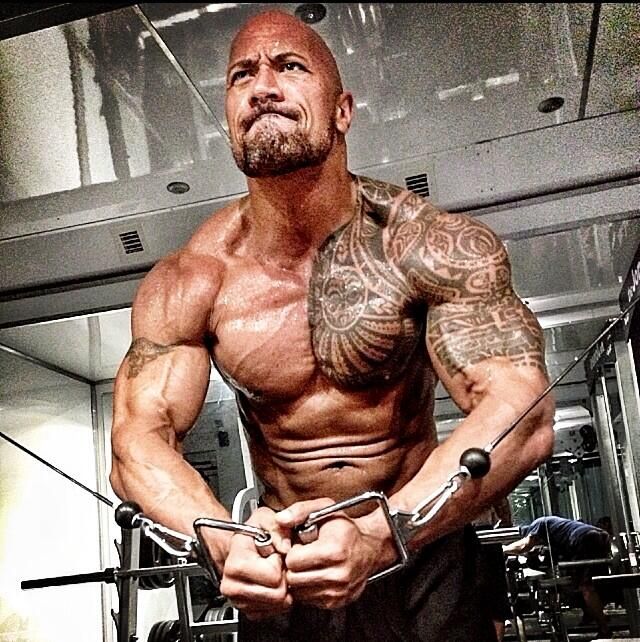The photograph depicts a highly muscular, pale-skinned man intensely working out in a well-equipped, upscale gym. He is shirtless, revealing bulging muscles and veins, with a detailed tribal Polynesian tattoo covering his left shoulder, bicep, and extending onto his chest. The man, bald and sporting a brown goatee, holds two silver handles attached to cables at waist level, clearly exerting himself. His serious expression conveys the effort he is putting into the exercise. The background features mirrors and a reflective ceiling, adding depth to the image, and various other gym machines are visible, including one being used by another person. Though his lower body is less visible, it appears he is wearing black shorts or pants. The gym's design includes clear glass elements, enhancing the space's sophisticated atmosphere.